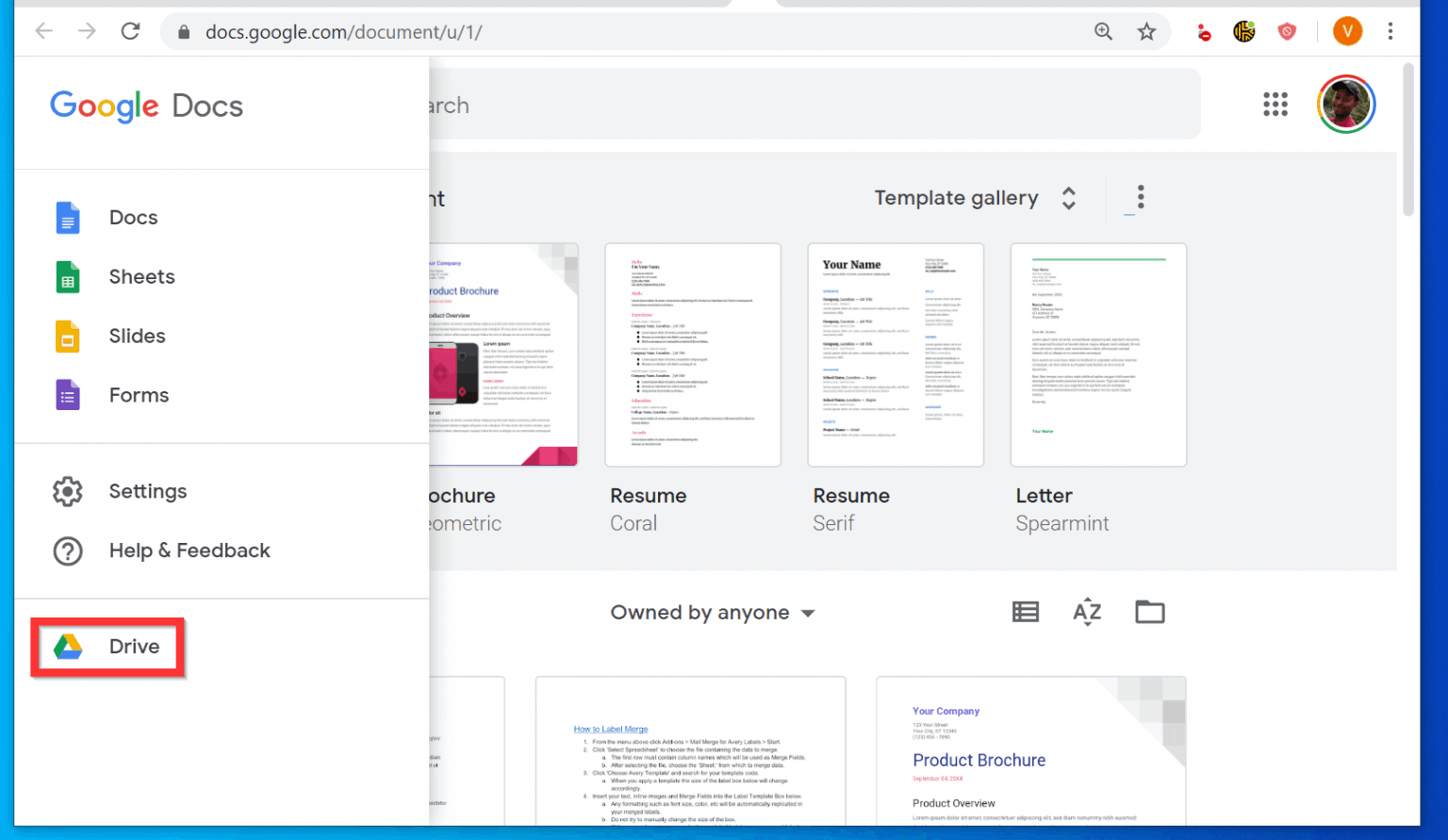The screenshot captures the Google Docs interface with various Google Workspace icons visible, including Docs, Sheets, Slides, Forms, Settings, Help, and Feedback. The Google Drive icon is prominent, highlighted by a red rectangle. There is an option to access the Template Gallery, though some elements are partially obscured by a popup window.

Within the popup window, templates for Google Docs are displayed, including brochures and resumes. Visible templates include:
- "OCHRE Resume"
- "Coral Resume"
- "Serif Resume" (noting that "Serif" denotes the font type)
- "Spearmint Letter"

In the top right corner of the interface, there is a user profile picture of a man appearing to be in his mid-20s. The browser's address bar shows the URL "docs.google.com/document/u/1/", with everything after "com" in gray text and the preceding part in black.